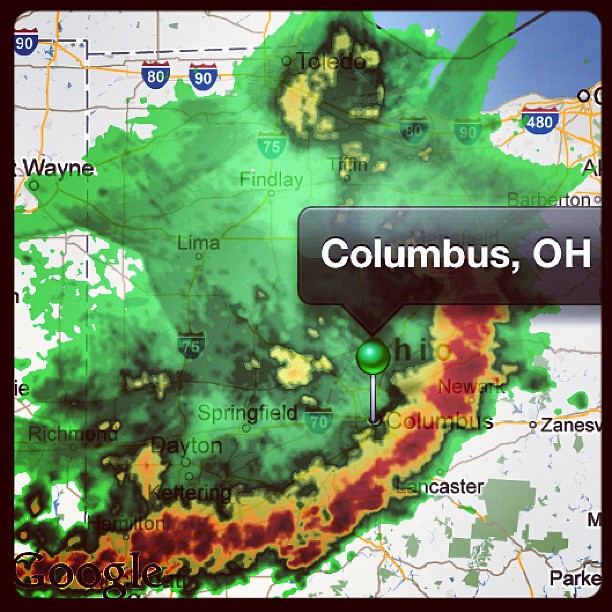The image is a detailed, digitally created weather radar map focusing on Columbus, Ohio. It showcases the current storm over the area, with a notable radar display of green, indicating a widespread weather system extending from Wayne to Springfield and Lancaster. A prominent band of heavy weather in red and orange is visible, highlighting severe conditions. The map features the name "Columbus, Ohio" in a gray bar with white text, like a pop-up pin, similar to Google Maps. Additionally, highway signs such as 80, 90, and 480 are marked, further identifying key areas affected by the storm. The radar screen uses a variety of colors, including dark green, light green, yellow, dark yellow, dark red, light red, blue, and shades of emerald and olive green, to represent different intensities of the weather system.